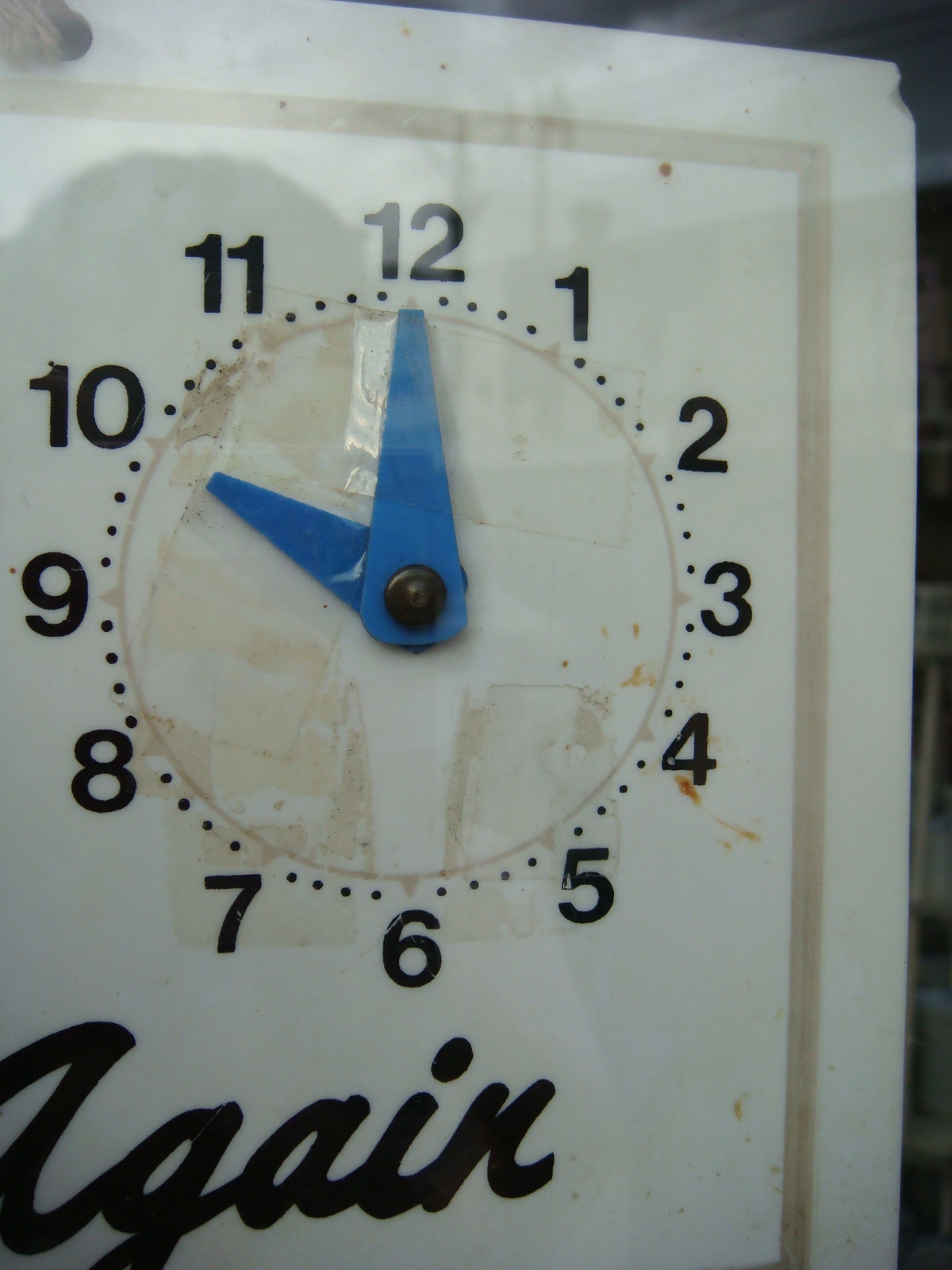The image is an extreme close-up of a clock face, from which the supporting structure is not visible, adding an element of mystery. The orientation of the image is slightly skewed, with a faint black line running vertically along the right edge and a small black triangular section protruding from the right corner, extending just past the midpoint of the top edge. The clock face itself is small and circular, featuring a golden-bronze hue.

Presenting a neat arrangement, black dots encircle the center to mark the time increments. Beyond these dots, black Arabic numerals from 1 to 12 are evenly spaced, indicating the hours. Encasing the entire clock face is a thicker band of the same golden-bronze color, possibly suggesting a rectangular frame around the clock, which blends seamlessly with the central circle.

The clock hands, shaped like elongated, rounded-off triangles with flattened tops, are dark blue in color. They point conspicuously to 10 o'clock, aligning snugly on the hour. In the bottom-left corner of the image, slightly cut-off yet discernible, is a bold, italic text that reads "again" in black ink. Although the full word is not completely visible, the letters "G-A-I-N" are clear, and the first "A" is partially shown as a capital letter, reinforcing the word "again."